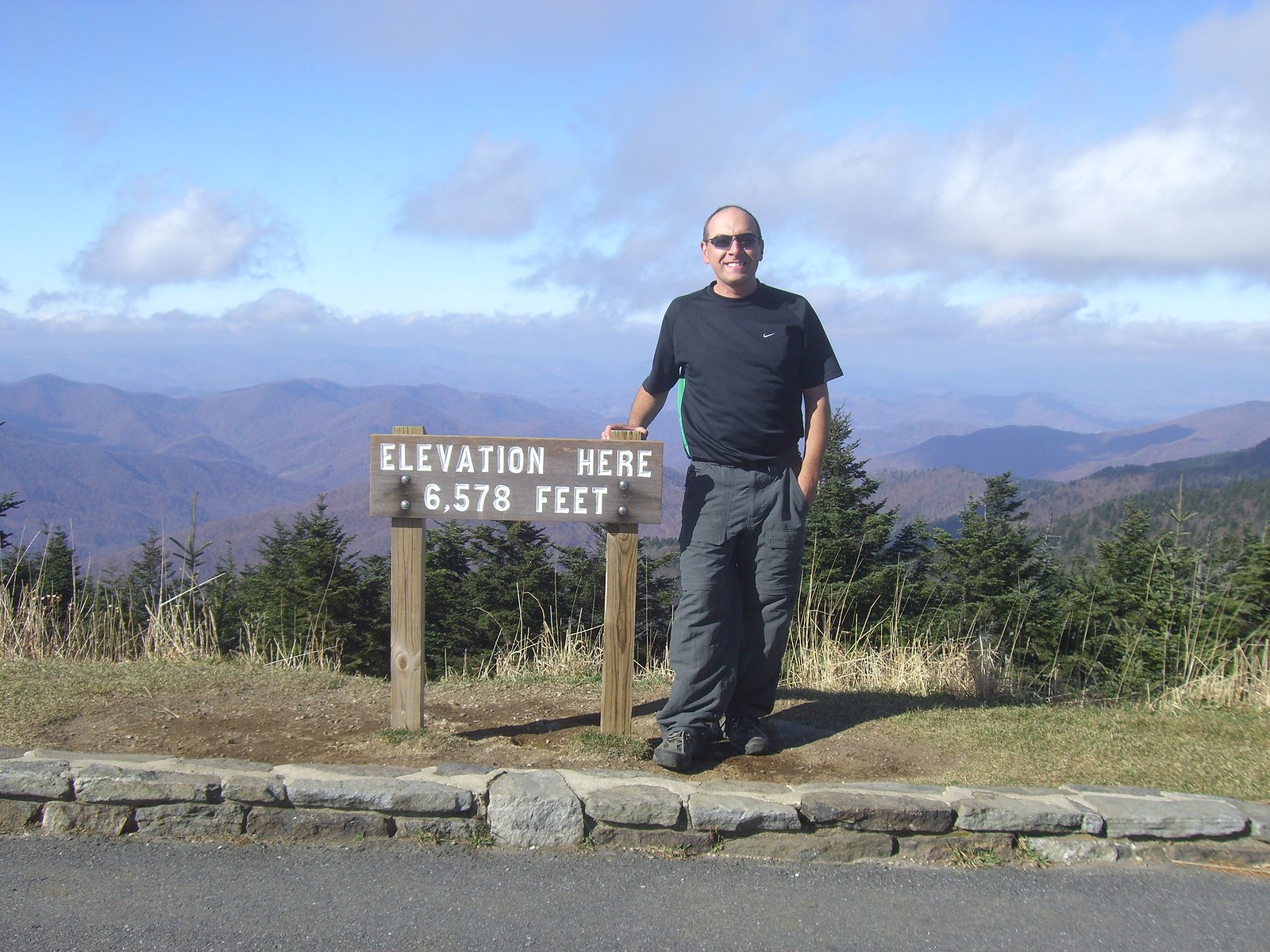In the photograph, a middle-aged Caucasian man is standing next to a wooden sign on the side of a road with a breathtaking view in the background. The man, who appears almost bald, is dressed in a black Nike shirt with a white logo on the right chest, gray pants, and gray shoes. He sports dark sunglasses and smiles at the camera. His left hand is casually placed in his pocket while his right hand rests on top of the wooden sign. The sign has white text that reads "Elevation 6,578 feet."

The setting is picturesque, with a stone curb bordering the asphalt road, leading to a dirt path that descends into a valley below. Behind the man, the background features an array of conifer trees, believed to be firs, stretching out over rolling hills and lower mountains, under a partly cloudy sky. This elevated vantage point provides a stunning view, with miles of pine trees and a scenic, mountainous horizon.